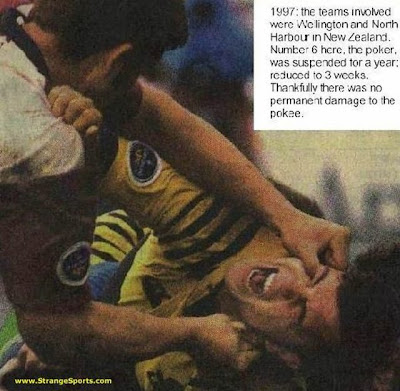This detailed image captures a heated moment during a rugby match in 1997 between Wellington and North Harbour in New Zealand. In the scene, a man wearing a dark reddish-brown and white jersey, identified as Number 6, is in the upper-left corner, aggressively holding down an opponent in a yellow jersey with black stripes, positioned in the lower-right corner. Number 6's arms are forcefully pinning the other man, his thumb cruelly digging into the man's eye, whose mouth is open in what appears to be a scream of pain. Both players have a blue and white patch on their sleeves. Above them, the corner text in a white box with black lettering provides context about the incident and its aftermath, noting that Number 6 received a suspension, initially for a year but later reduced to three weeks, without causing permanent damage to his opponent. The bottom left corner also has a small yellow text indicating www.strangesports.com, likely the source of the image. The struggle and intensity are palpable, set against an indeterminate background typical of an outdoor sports field.